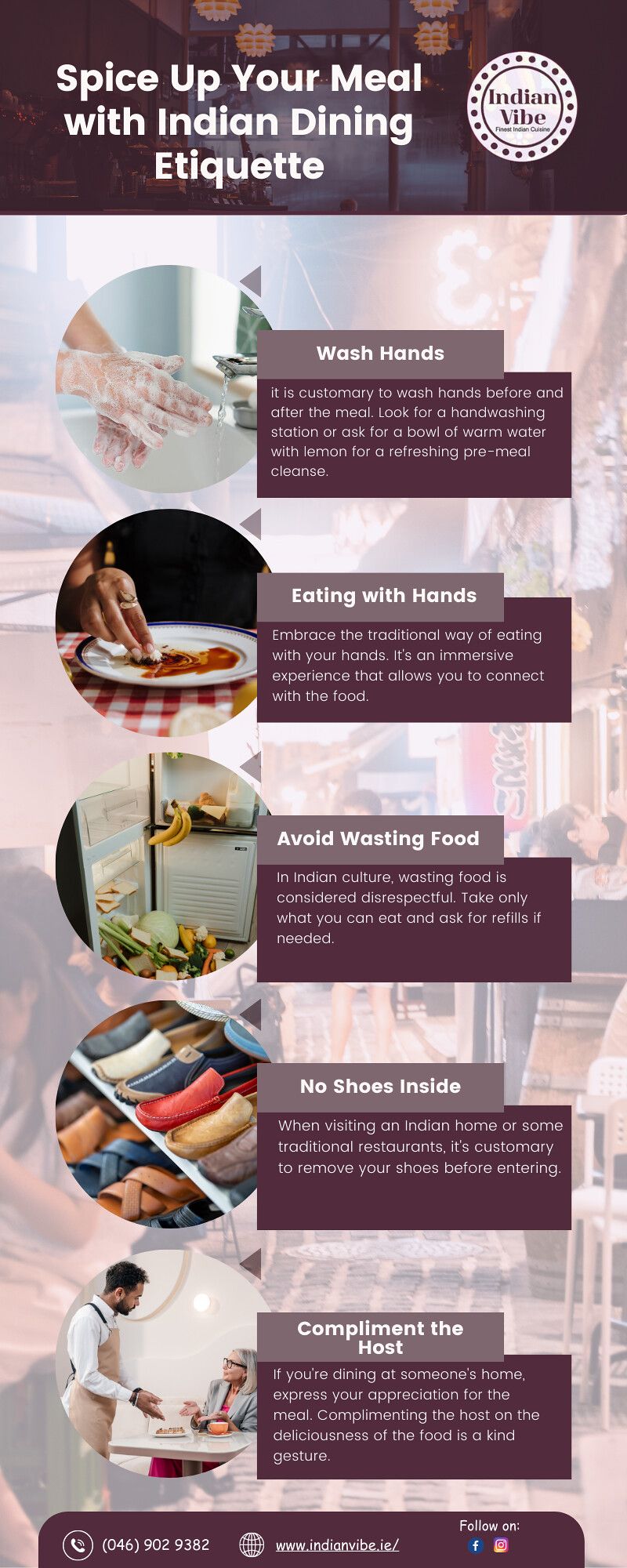The image displays a descriptive pamphlet titled "Spice Up Your Meal with Indian Dining Etiquette," featuring a burgundy banner at the top with white text. Centered within a white circle on the banner is burgundy text reading "Indian Vibe." The background showcases scenes of people dining at various restaurants. The foreground is filled with burgundy rectangles containing white text and corresponding images, explaining essential dining practices. The first rectangle depicts someone washing their hands in a sink, with text advising to wash hands before and after meals, suggesting a hand washing station or a bowl of warm water with lemon. The second rectangle shows a person eating with their hands, emphasizing the custom of eating with hands. The third rectangle features bananas in a fridge, underlining the importance of avoiding food waste. The fourth displays shoes on a rack, reminding viewers to leave shoes outside. The fifth illustrates a host speaking to a guest, encouraging compliments to the host. At the bottom, contact details including a phone number, a website, and social media links for "Indian Vibe" are provided.